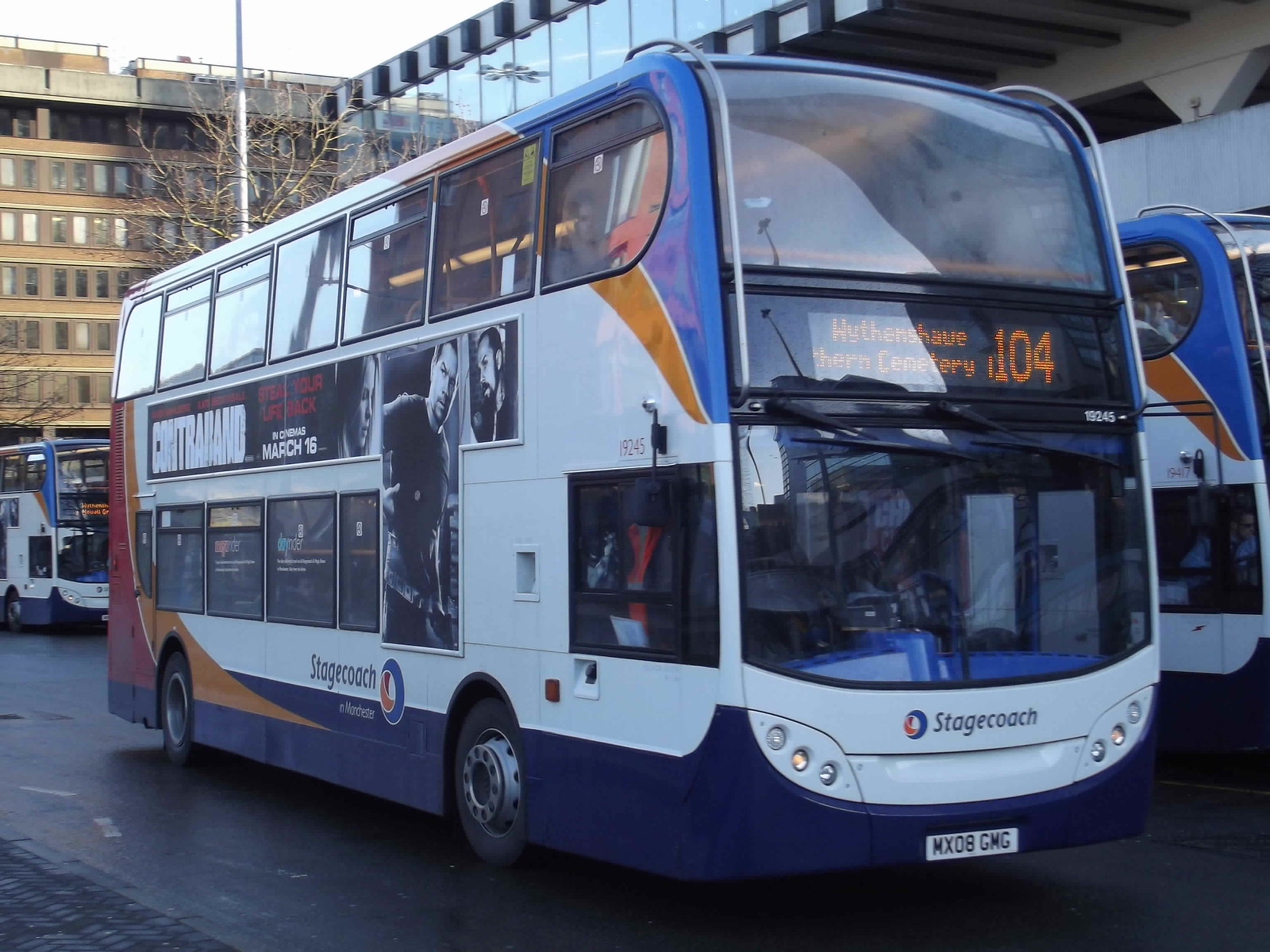In the wide rectangular image, a white double-decker bus with a red, gold, and blue pattern is captured traveling diagonally down a dark gray road, heading to the right. The front of the bus prominently displays "104 Wythenshawe Northern Cemetery" in bright orange lit letters. An advertisement on the bus features a black-and-white picture of three people with the text "Contraband, in cinemas March 16th" in bold white font. The lower part of the bus includes the branding "Stagecoach." Surrounding the main bus, there are other buses visible on the same street. The backdrop reveals a bustling cityscape with residential buildings, stores, and tall structures with numerous glass windows, suggesting an urban environment that may be located in the UK, given the double-decker bus style.